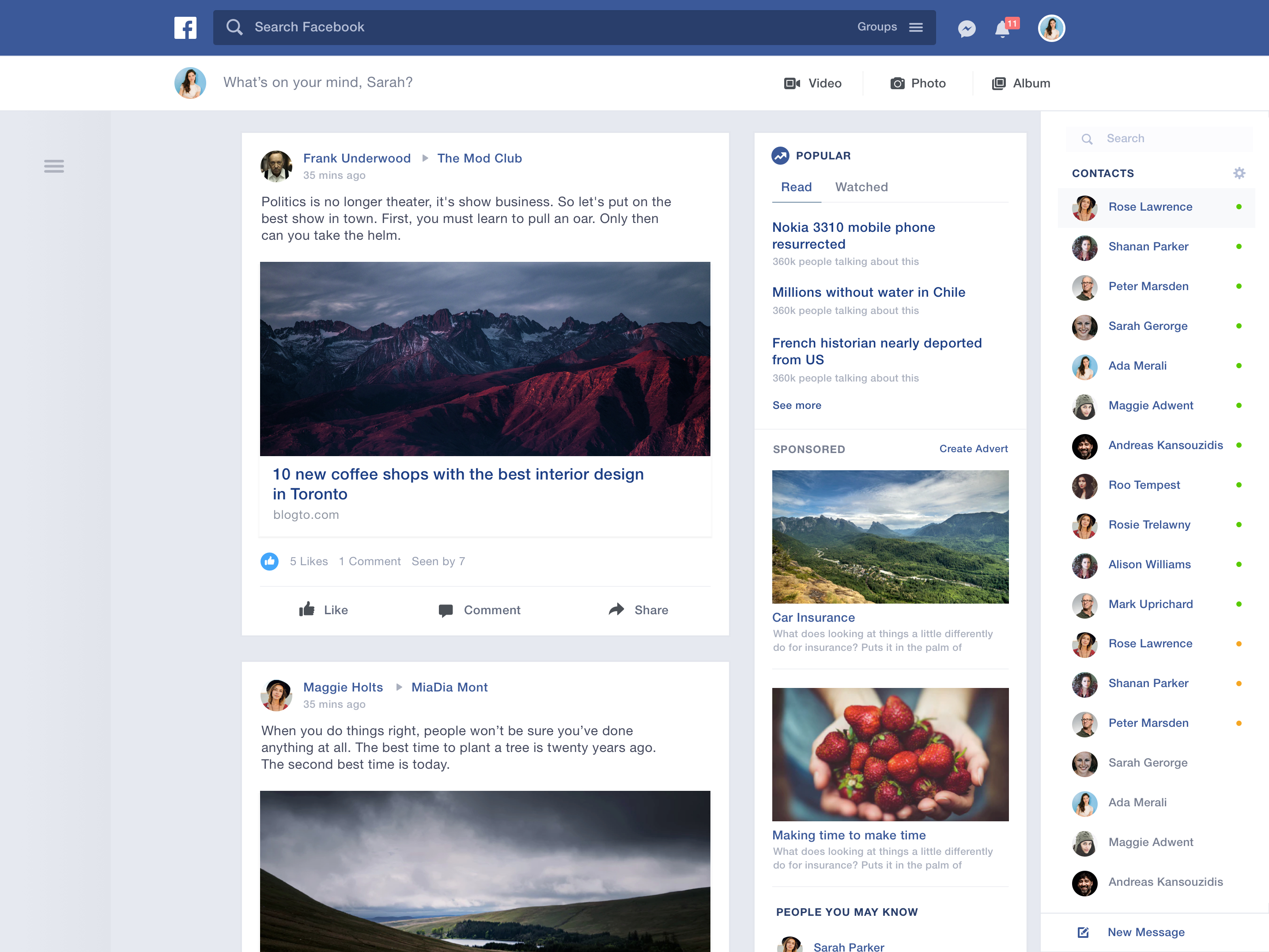The image depicts a detailed view of a Facebook page interface. At the very top, a blue ribbon spans the width of the screen, featuring the iconic white "F" Facebook logo and an adjacent search bar for navigating the site. On the far right, the word "Groups" indicates that the user is exploring the group's section. Also visible are icons for Messenger, with an alert indicating 11 new messages, and the user's profile picture within a circle. 

Below the ribbon, the user’s profile picture appears again against a white background, with the prompt "What's on your mind, Sarah?" inviting her to type a status update. Adjacent to this text input area are icons for sharing a video, photo, or album.

The timeline includes a post from Frank Underwood associated with the "Mod Club," displaying an image of a mountain range split into blue and red hues. Frank's caption reads: "Politics is no longer theater. It's show business. So let's put on the best show in town. First, you must learn to pull an oar. Only then can you take the helm." 

Further down, a highlighted text snippet promotes an article titled "10 new coffee shops with the best interior design in Toronto," and additional posts from various users follow. On the far right side of the page, a list of the user’s contacts suggests that the Messenger app is currently active.